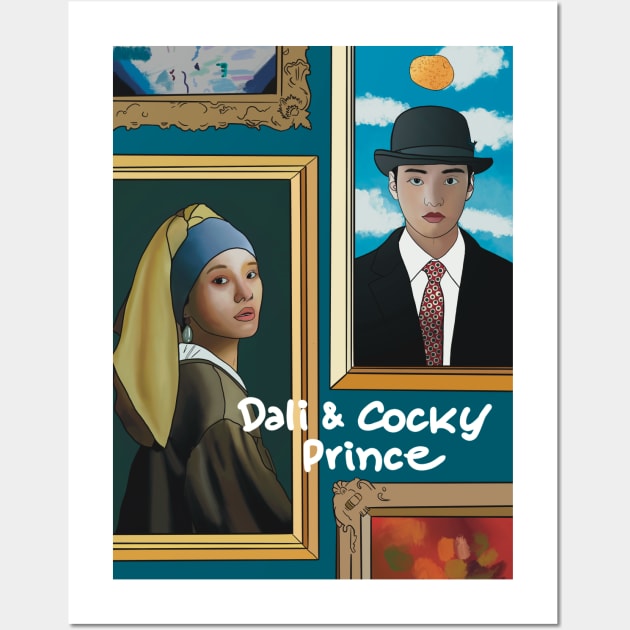The image is a detailed illustration depicting two framed portraits set against a blue background, both bordered by intricate gold frames. The left portrait features a woman styled similarly to the "Girl with a Pearl Earring," but with distinctive differences: she has tanner skin, is wearing a blue and yellow cowl, a brown gown, and a prominent silver earring, and is posed facing left while looking towards the camera with a pensive expression. The right portrait showcases a person in a formal outfit consisting of a blue suit jacket, a white shirt, a red patterned tie, and a black hat. They are standing against a backdrop of a blue sky with an orange floating above their head and gaze directly at the viewer. The text "Dolly and Cocky Prince" is elegantly displayed in white cursive across the forefront of the illustration, uniting the visual elements.